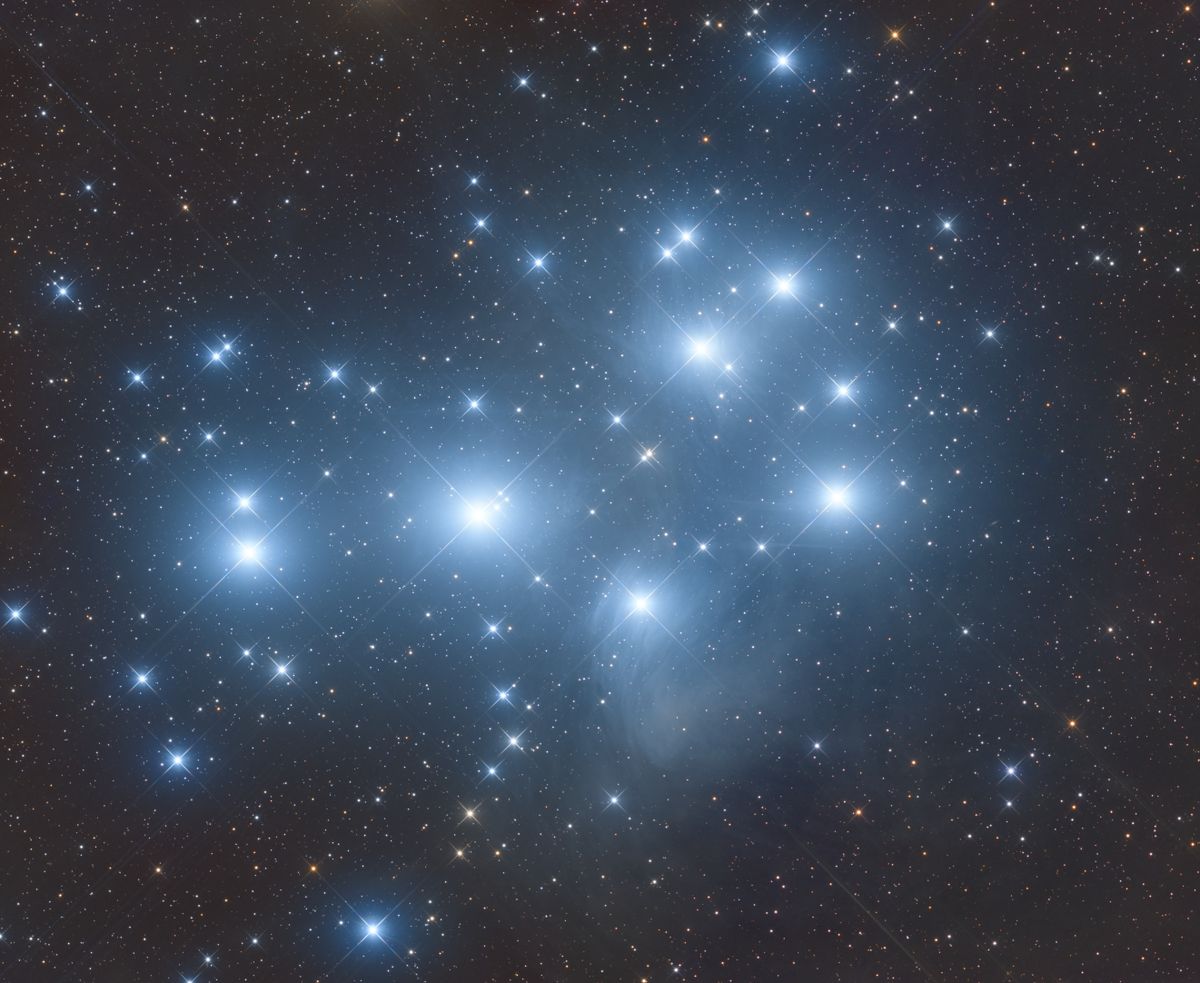This high-resolution, square image captures the expanse of a dark night sky, filled with countless stars that appear as tiny pinholes against the black backdrop of space. A significant focal point is the dense star cluster situated slightly right of the center, featuring about fifty stars. Within this cluster, several bright white stars dominate, their intense glow creating faint lens flare patterns that resemble refracted light. This central area is tinged with a subtle blue hue, enhancing the overall luminosity.

Interspersed among the predominantly white stars, you can spot a few that emit orange, yellow, and blue hues. One particularly bright star, the most luminous in the image, is positioned just left of center. Below it, a string of slightly smaller but still prominent stars forms a downward and leftward trail, terminating near another bright star at the image's lower left edge.

Additional bright stars are scattered across the image, including a pair in the upper right quadrant, a few more tiny ones in the lower right, and clusters of faint stars in the upper left and right corners, as well as the lower middle area. This striking image, likely computer-generated or captured via a telescope, beautifully showcases the varied brilliance and distribution of stars in the night sky.